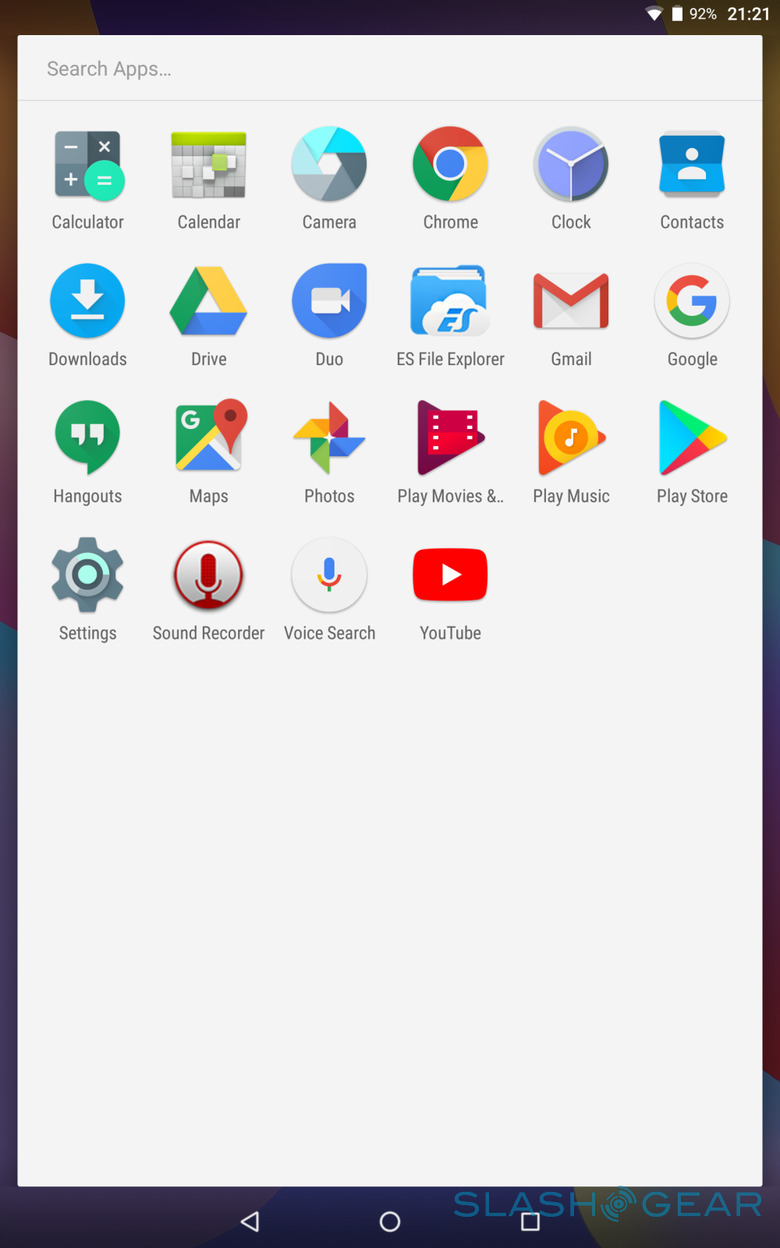The image shows the screen of a mobile device, likely a phone or tablet. At the top right corner, the nearly full Wi-Fi signal icon and a battery icon at 92% are displayed next to the time, which is 21:21. The background of the screen appears slightly artistic. 

In the foreground, a large white rectangle overlays the background, and at the top left of this rectangle is the text "Research apps..." followed by a gray line. Below this line, there are several rows of app icons arranged in a grid format. 

The first row features the following apps with their respective icons: Calculator, Calendar, Camera, Chrome, Clock, and Contacts. The second row includes: Downloads, Drive, Duo, File Explorer, Gmail, and Google. The third row showcases: Hangouts, Maps, Photos, Play Movies & TV, Play Music, and Play Store. In the final row, the apps displayed are: Settings, Sound Recorder, Voice Search, and YouTube. 

Below these rows of app icons, there is a large blank white space extending downwards. At the bottom edge of the screen, three classic navigation buttons are visible: the left-pointing triangle for 'Back,' the circle for 'Home,' and the square for 'Recent Apps.'

This detailed description captures the layout and elements present in the screenshot of the mobile device screen.